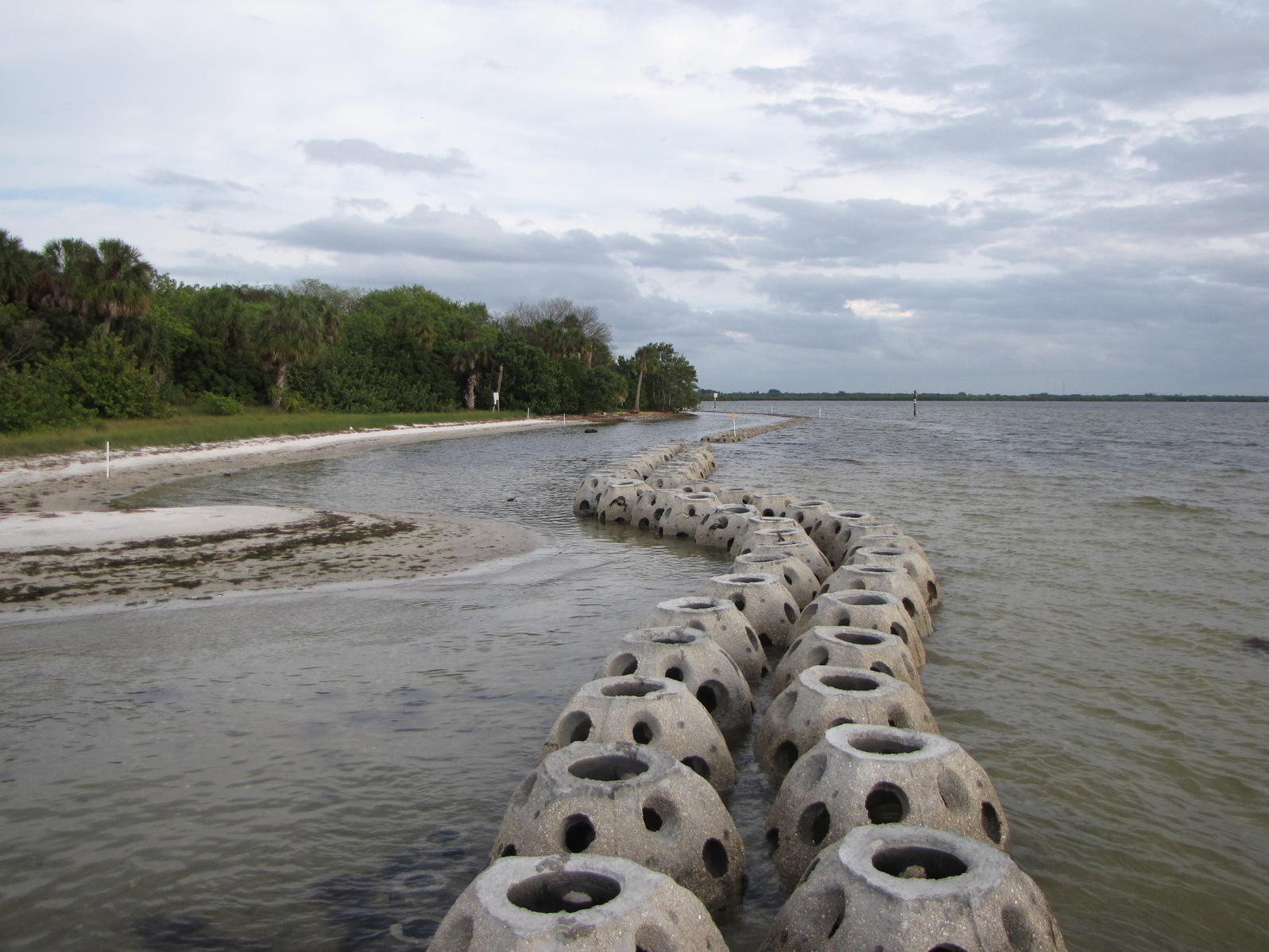This photograph depicts a picturesque yet somewhat desolate beachfront that seems to be part of a deserted island. The focal point is the water, which has a murky green hue, contrasting with the typical blue we associate with tropical paradises. Two rows of large, hollow, cement blocks, reminiscent of oversized bowling balls with finger holes, stretch from the foreground into the distance, possibly serving an environmental function like erosion control. These cement pieces are meticulously aligned, curving to match the shoreline's natural shape.

To the left side of the image, dense clusters of tall, rich green trees rise from a patch of grass that puzzlingly extends close to the water's edge, an unusual sight for a beach typically bordered by sand or rocky outcrops. The shoreline itself consists of light-colored brown sand, transitioning into a shallow water area where these cement structures are positioned. The scene is devoid of any human activity or boats, enhancing its isolated atmosphere.

Above, an overcast sky filled with light gray and bluish clouds forms a somber canopy over the scene, adding a layer of melancholy to the landscape. The photograph, with its lack of identifying marks or people, evokes a sense of mystery and tranquil abandonment.